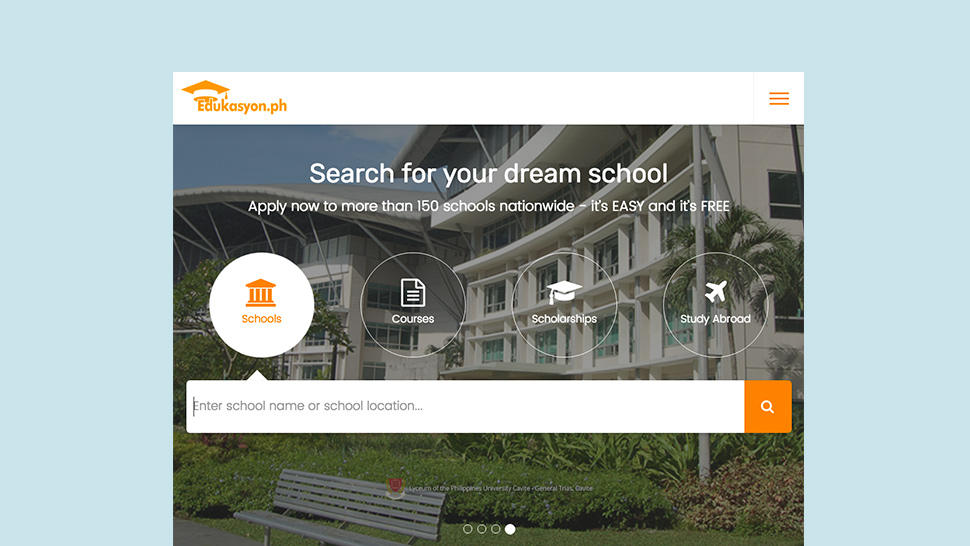On a serene pale pastel blue background, the image portrays a sophisticated website interface. On the left side, a white header is prominently displayed featuring an orange logo with a graduation hat underneath. The text "edukasya n oron.ph" is elegantly written. Towards the far right of the header, a light gray divider segues into three orange lines, signifying a drop-down menu.

The main content area showcases a visually appealing background image of what appears to be a luxurious hotel or corporate building, surrounded by abundant vegetation and various bushes. The backdrop includes a vivid blue sky with delicate, wispy clouds to the left.

In the center of the website, four distinct circular options are visible. The first option, labeled "Schools," is highlighted in white indicating it is selected, and features an orange school building icon. Below this, a search field in gray prompts with the text "Enter school name or school location..."

Next to "Schools" is the "Courses" option with a transparent background, showcasing a white piece of paper icon with three lines. Following this is "Scholarships," represented by a white graduation cap icon, also on a transparent background. The last option, "Study Abroad," features a white plane icon with the label beneath it, similarly on a transparent background.

Below the search area, a gray bench is placed, with a red icon situated toward the right end of the bench, adding a subtle pop of color to the scene. The detailed elements together create a cohesive and visually engaging web page layout.